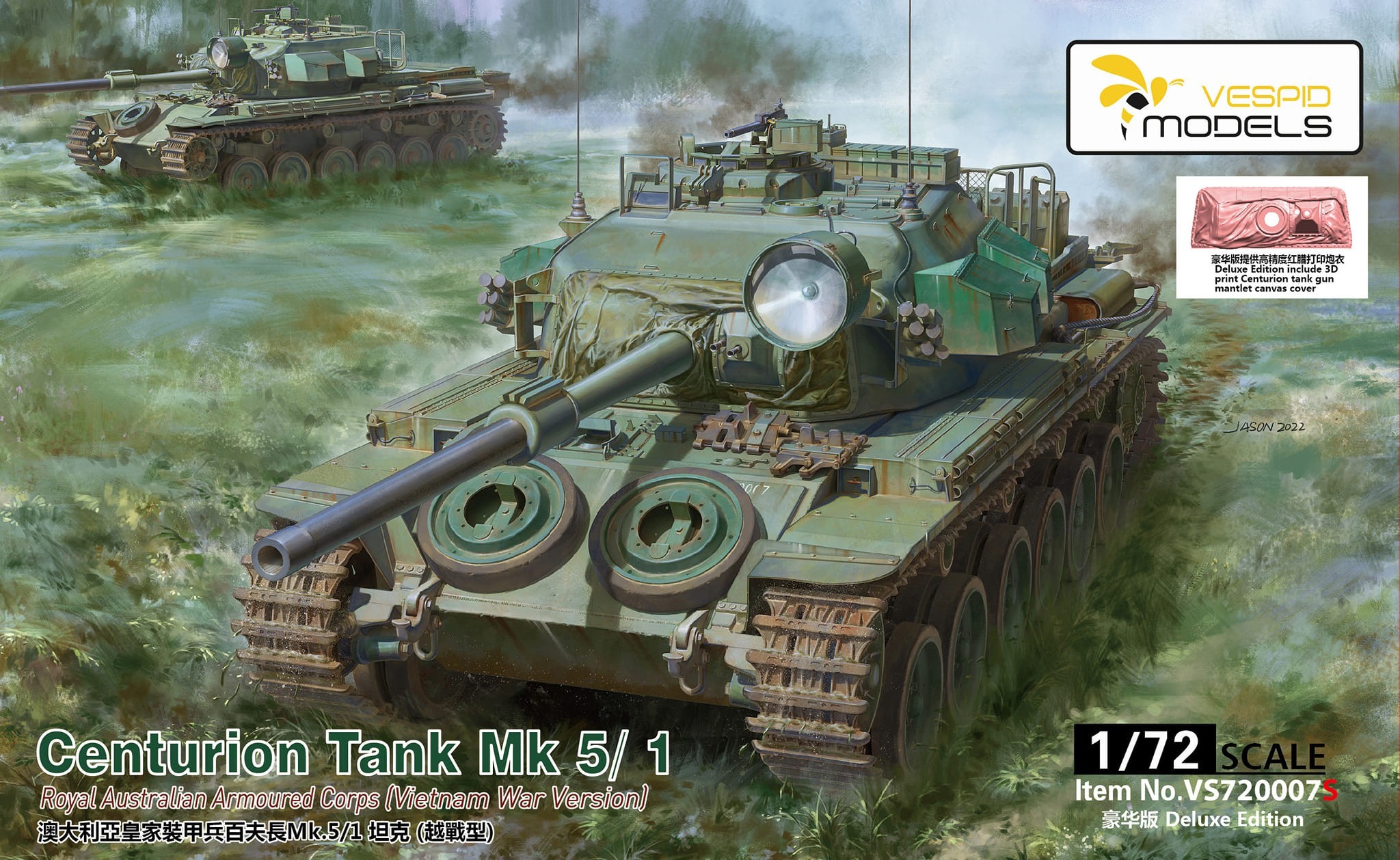The cover art for this 1/72 scale model kit box by Vespid Models features a detailed color illustration of a green Centurion Tank MK5-1 used by the Royal Australian Armored Corps during the Vietnam War. Dominating the center, the main tank is depicted in a diagonal position with its gun barrel slightly pointed towards the left. Another smaller tank appears in the background at the top left, with dark smoke billowing from its rear, set against a misty backdrop with green, blue, and gray tones, suggesting a smoky and possibly aquatic environment with greenish-brown water. In the upper right-hand corner, encased in a white box, is a pink canvas cover associated with the Deluxe Edition, specifying the inclusion of a 3D printed Centurion Tank Gun Mantlet Canvas Cover. The top of the illustration is marked with the Vespid Models logo featuring a stylized wasp or hornet. Additional text and small white boxes with information and Chinese writing are scattered around the image. The bottom right specifies this as a Deluxe Edition item, numbered VS720007S, while the bottom left reiterates the model and scale details: Centurion Tank MK5-1, Royal Australian Armored Corps, Vietnam War version. The name Jason 2022 is noted slightly right of center.